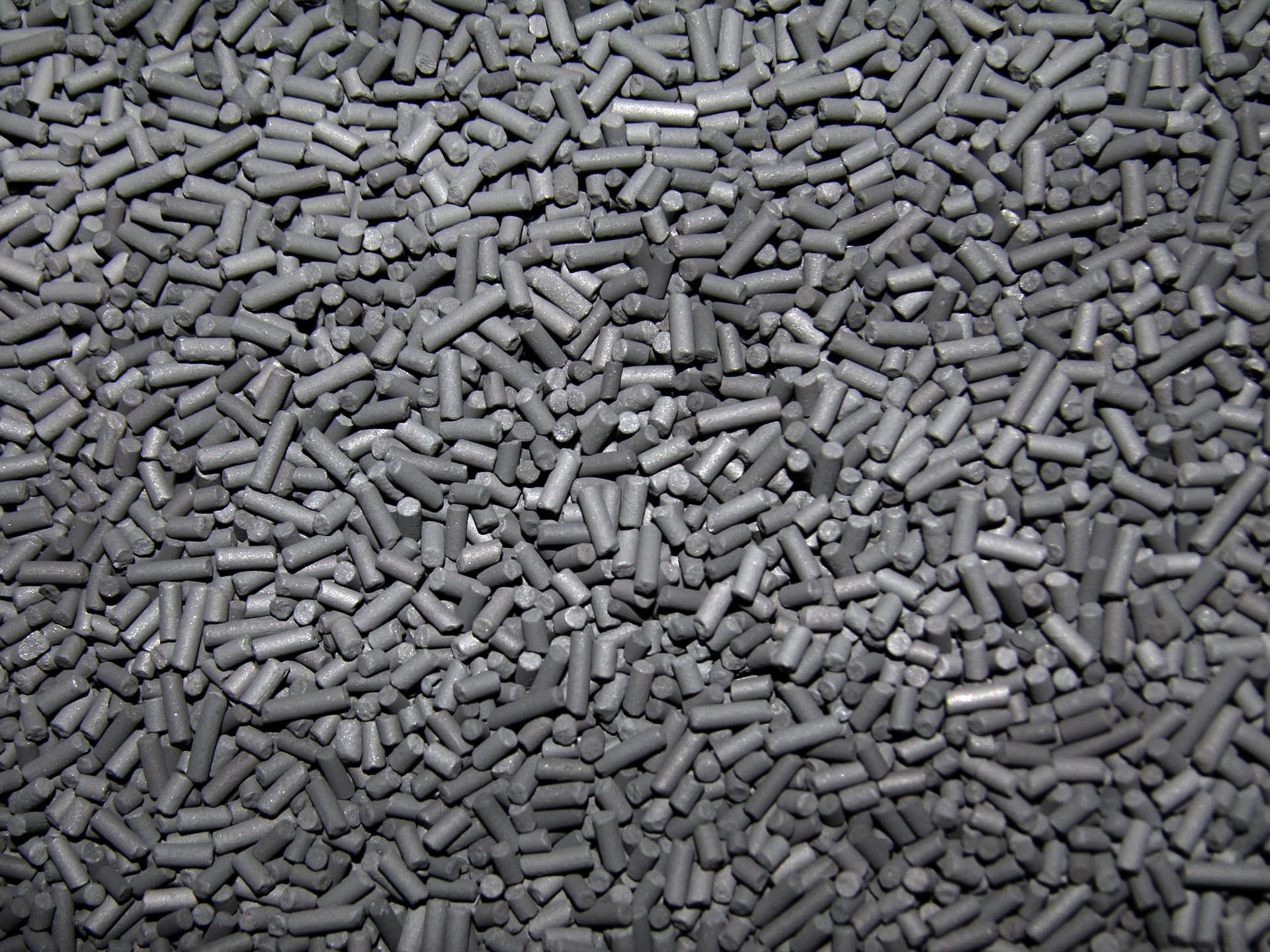The photograph features a detailed close-up of an entire surface covered with small, cylindrical objects that resemble pellets or perhaps pieces of chalk. The scene is predominantly monochromatic, with varying shades of gray—from light to dark—and even black. These cylindrical pieces, which are uneven in size and condition with some chipped or broken, are scattered randomly, creating a textured, chaotic pattern. The image has a slight vignette, darkening towards the edges, highlighting the central cluster of these pellets. The overall effect is a visually dense, intricate spread of these grayish cylinders, with the close-up perspective emphasizing their small, roughly pill-sized dimensions.